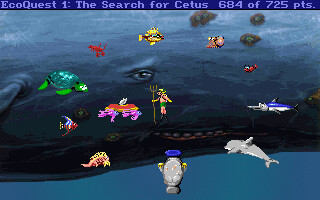This image appears to be a screenshot or still from the video game "EcoQuest 1: The Search for Cetus," displaying a vibrant and nostalgic 80s-style design. Dominating the background is a massive sea creature that resembles a whale, with a prominent eye positioned centrally within the frame. Beneath the eye, a man holding a pitchfork stands, seemingly part of the game's narrative. Surrounding this focal point are pixelated, cartoonish sea creatures, including fish, dolphins, and a striking bright green turtle, all rendered in a colorful palette reminiscent of the rainbow. A purple banner strip at the top of the image reads, "EcoQuest 1: The Search for Cetus, 684 of 725 PTS," indicating the player's score. The whale's surface shows some pixelation, and there are small brown landmarks atop its head, adding detail to the underwater scene.